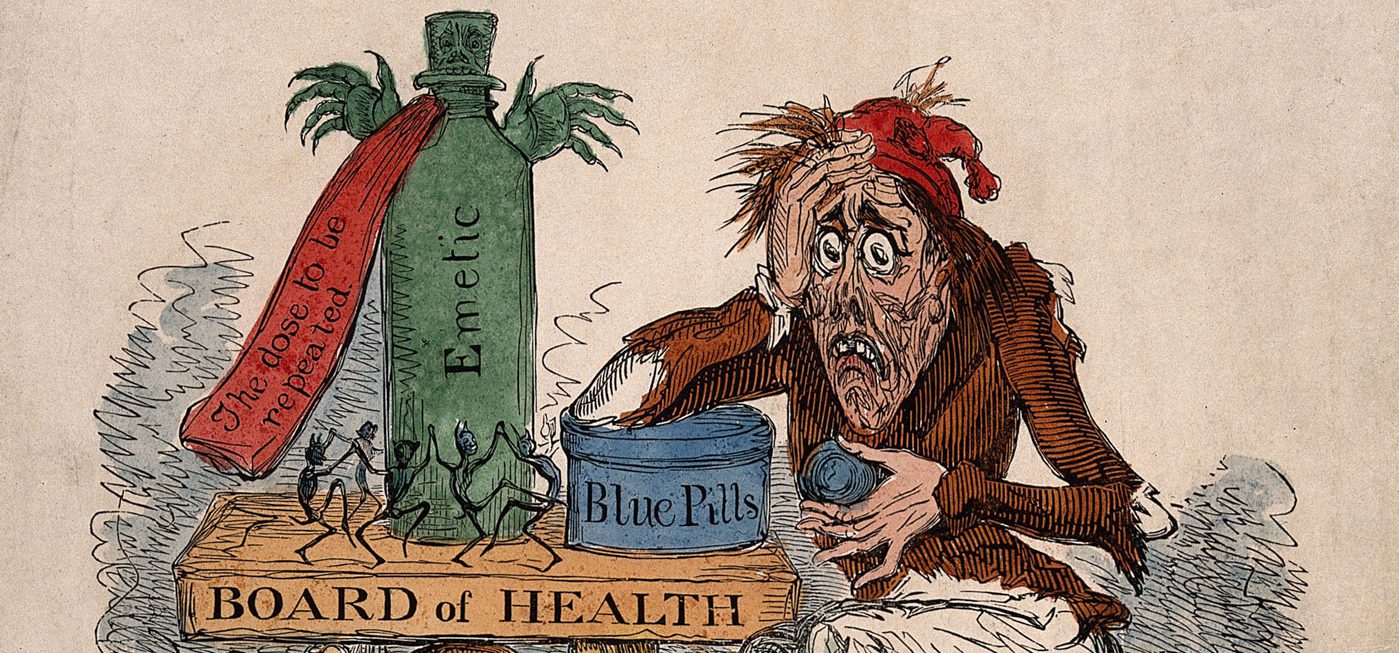In this detailed old-fashioned cartoon, we observe a very nervous, worried man sitting at a table, showcasing a clear sense of satire. With wild hair, bulging eyes, and wearing tattered clothing consisting of a brown shirt and a red nightcap, his distressed demeanor is palpable. The man’s elbow rests on a container labeled "blue pills" in blue text. Positioned on the table, which is marked "Board of Health," is a green bottle labeled "emetic," featuring a ribbon that states "this dose to be repeated." The man’s hand clasps his forehead, enhancing his appearance of shock or psychedelic distress, while the emetic bottle bears a skull-adorned cap with small hands extending from it, adding to the eerie, cautionary atmosphere of the image.